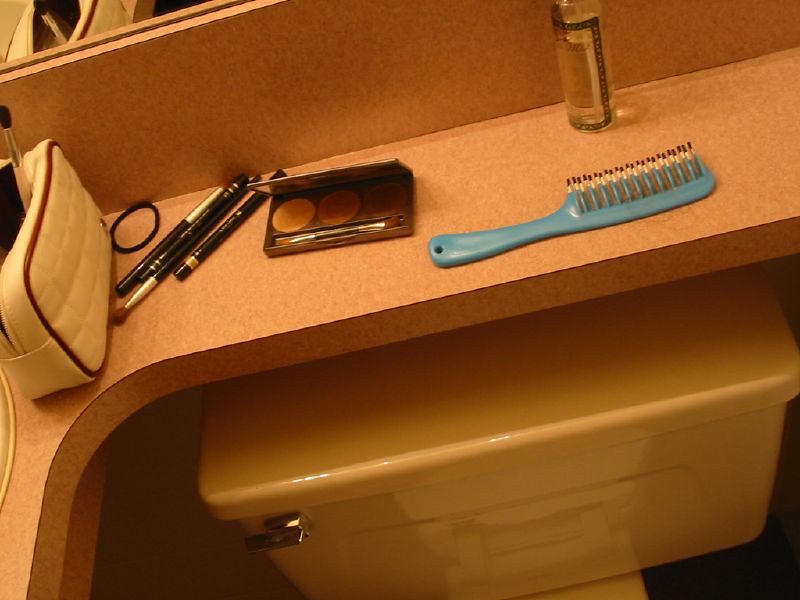The image captures an overhead view of a peach-colored, dotted L-shaped shelf situated above a white, rectangular toilet with a metallic handle. The rounded edges of the shelf add a soft touch to the bathroom decor. On the left side of the shelf, a rectangular white purse with a red band prominently rests. Beside the purse is a black hair tie, lying near a set of makeup brushes with black handles, silver tops, and brown bristles. An open makeup blush case, featuring three circular blush compartments, sits adjacent to the brushes. Close by, a blue comb with white teeth is slightly turned on its side. Above the comb, a transparent bottle with a green and white label adds to the assortment of items. The pristine white toilet below forms a stark contrast to the colorful and varied items on the shelf, creating an interesting vignette of everyday bathroom organization.